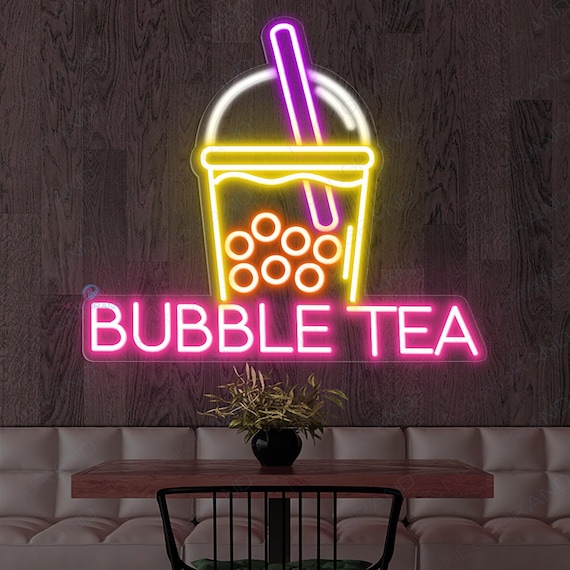In a cozy, chic bubble tea shop, a striking neon sign dominates a gray wood-paneled wall behind a sleek table and comfortable seating. The neon sign features vibrant colors: a yellow-outlined cup brimming with orange circles representing the liquid, topped with a white bubble and a purple straw. Underneath the cup, "Bubble Tea" glows in bright pink neon letters. The seating arrangement consists of a cream-colored, padded bench that runs along the length of the wall, offering a comfortable spot for patrons. A narrow wooden table, supported by a sturdy black metal post, sits in front of the bench. At the center of the table, a black vase holding a green plant adds a touch of nature to the modern setting. The contemporary elements and the vivid neon sign create an inviting and lively atmosphere, perfect for enjoying a delicious bubble tea.